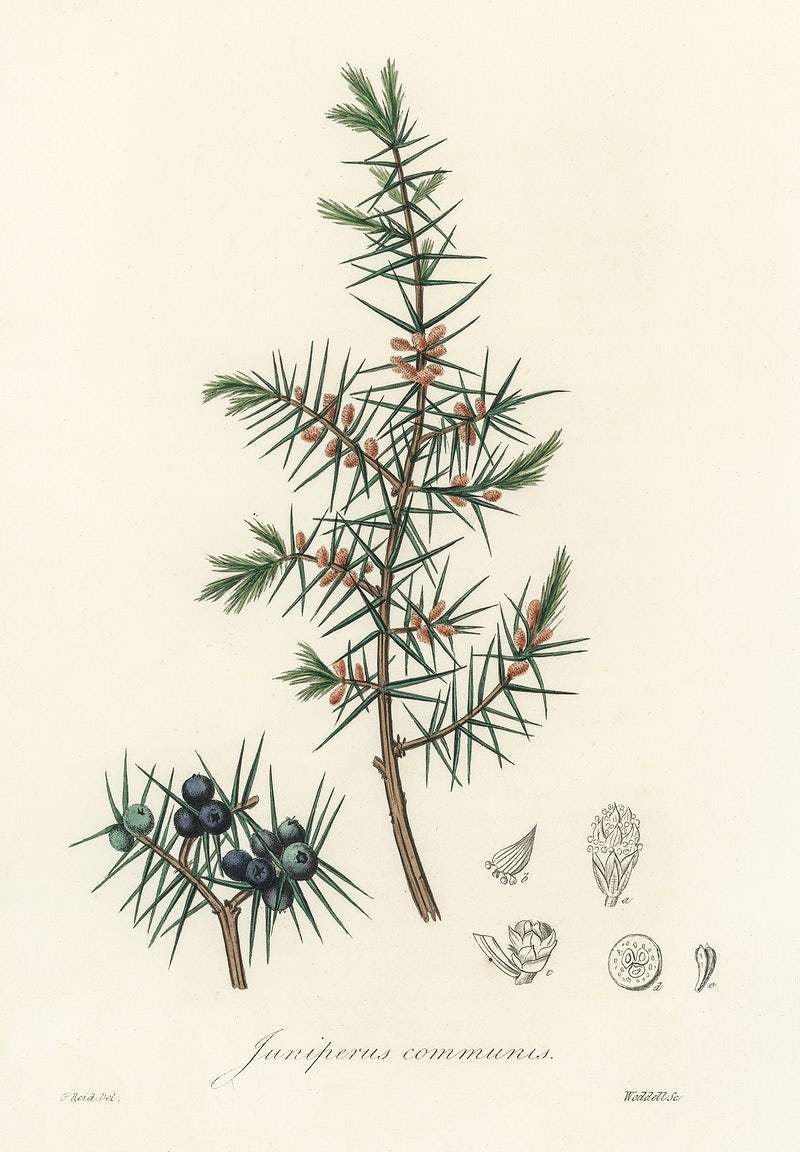This elegant vintage-style illustration showcases Juniperus communis, highlighted against a creamy off-white background. Dominating the center is a tall, slender branch depicted in light brown, adorned with dark green, jagged pine needles and numerous small, brown cones or nut-like structures scattered throughout. To the left, a smaller branch mirrors the central one but features clusters of berries in varying shades of purplish-blue, resembling blueberries. These branches have additional green needle-like leaves amidst the berries. 

The illustration also includes detailed pencil sketches on the bottom right, comprising several close-up studies of leaves and a small circular motif. At the illustration's base, a faint light blue cursive inscription reads "Juniperus communis," along with some additional, less legible text, possibly an artist's signature or further botanical notes. To the right of the branches, there are delicate line drawings displaying the different stages of a budding flower and a cross-sectional view, adding to the scientific and educational charm of this botanical artwork.